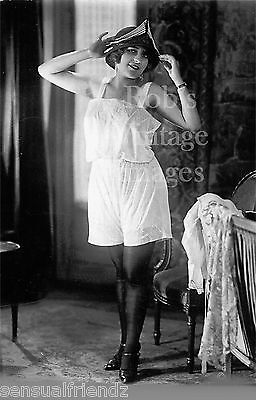The black-and-white vintage photograph, stamped with "Rob's Vintage Images" at the top and the barely visible "Sensual Friendz" at the bottom, captures a young, smiling woman posing gracefully in her bedroom. She is dressed in a white romper with thick straps, resembling period-specific camisole and shorts that exude a risqué allure for the time. Her ensemble is completed with black stockings and black strapped high heels. She has a sleek bob haircut and dons a V-shaped crown tiara, which she adjusts with her hands raised to her head. The room, framed by thick, ornate curtains in the background, features an upholstered chair to her right and what appears to be the end of a bedframe to her left. In an elegant gesture, she tilts her head slightly as her joyful expression suggests a playful yet poised demeanor, embodying the charm of the flapper era.